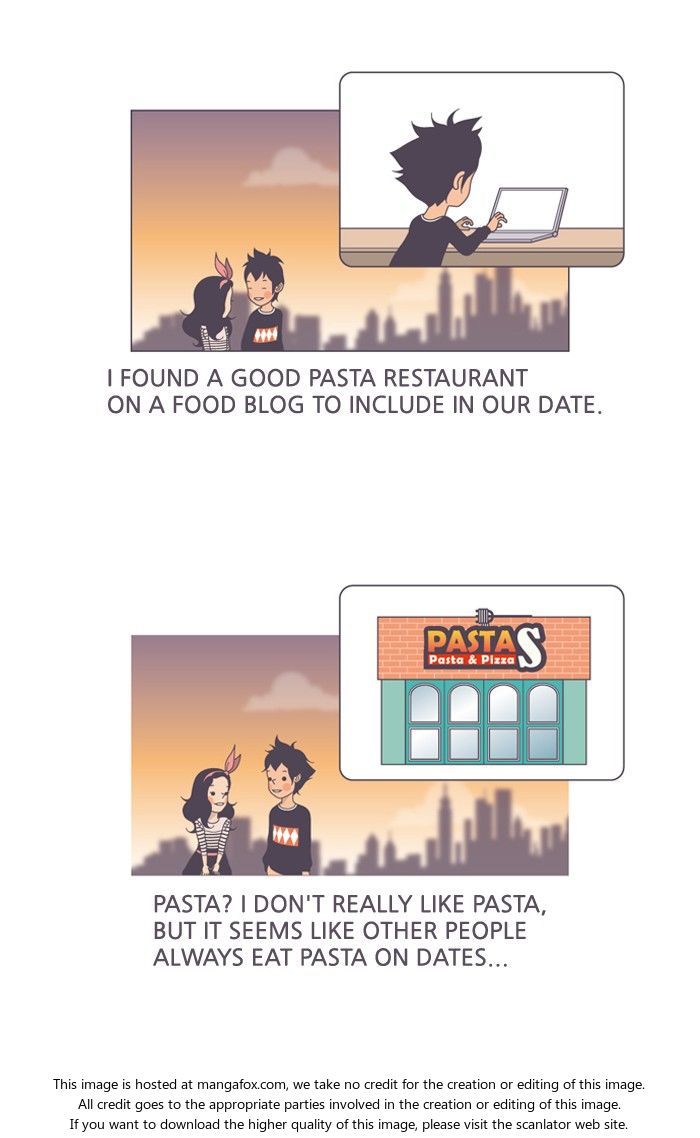The image consists of two vertically stacked illustrations from what appears to be an online comic strip, set against a muted peach and red cityscape with an orange and brown skyline. Both panels feature two dark-haired, anime-style cartoon characters—a male and a female distinguished by the girl's pink bow. In the top panel, the male character is at a laptop, with a thought bubble that reads, "I found a good pasta restaurant on a food blog to include in our date." A smaller window in this panel shows him working on his laptop. In the bottom panel, the female character faces the viewer, responding with, "Pasta, I don't really like pasta, but it seems like other people always eat pasta on dates." There’s a notable detail in both panels of a sign in the background that reads "Pasta and Pizza." The overall color scheme features muted, peachy tones mixed with soft reds. The image appears to be hosted on magnafox.com, which notes that they take no credit for its creation, directing users to the Scanlator website for higher quality downloads.